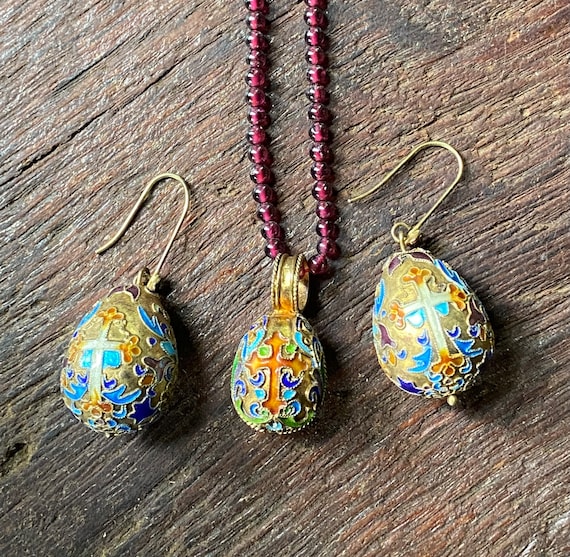A top-down photographic image presents an antique matching jewelry set elegantly arranged on a weathered oak table. The worn, textured surface features rich tones of dark and lighter browns interspersed with reddish hues, accentuating the vibrant colors of the jewelry. The set includes a pair of earrings flanking a pendant necklace, all featuring a distinctive mini Fabergé egg design. Each egg-shaped piece showcases a striking turquoise background adorned with intricate gold patterns and darker orange highlights. Central to each piece is a prominent crucifix, with the earrings displaying gold crosses and the pendant a contrasting burnt orange cross. The earrings, equipped with gold hooks for pierced ears, mirror the pendant's design. The pendant is affixed to a partially visible beaded maroon chain, completing the necklace. The meticulous detailing suggests a tactile, three-dimensional quality, making the jewelry appear raised and textured. This composition suggests an intentional photographic setup, possibly to highlight the intricate craftsmanship for potential sale.